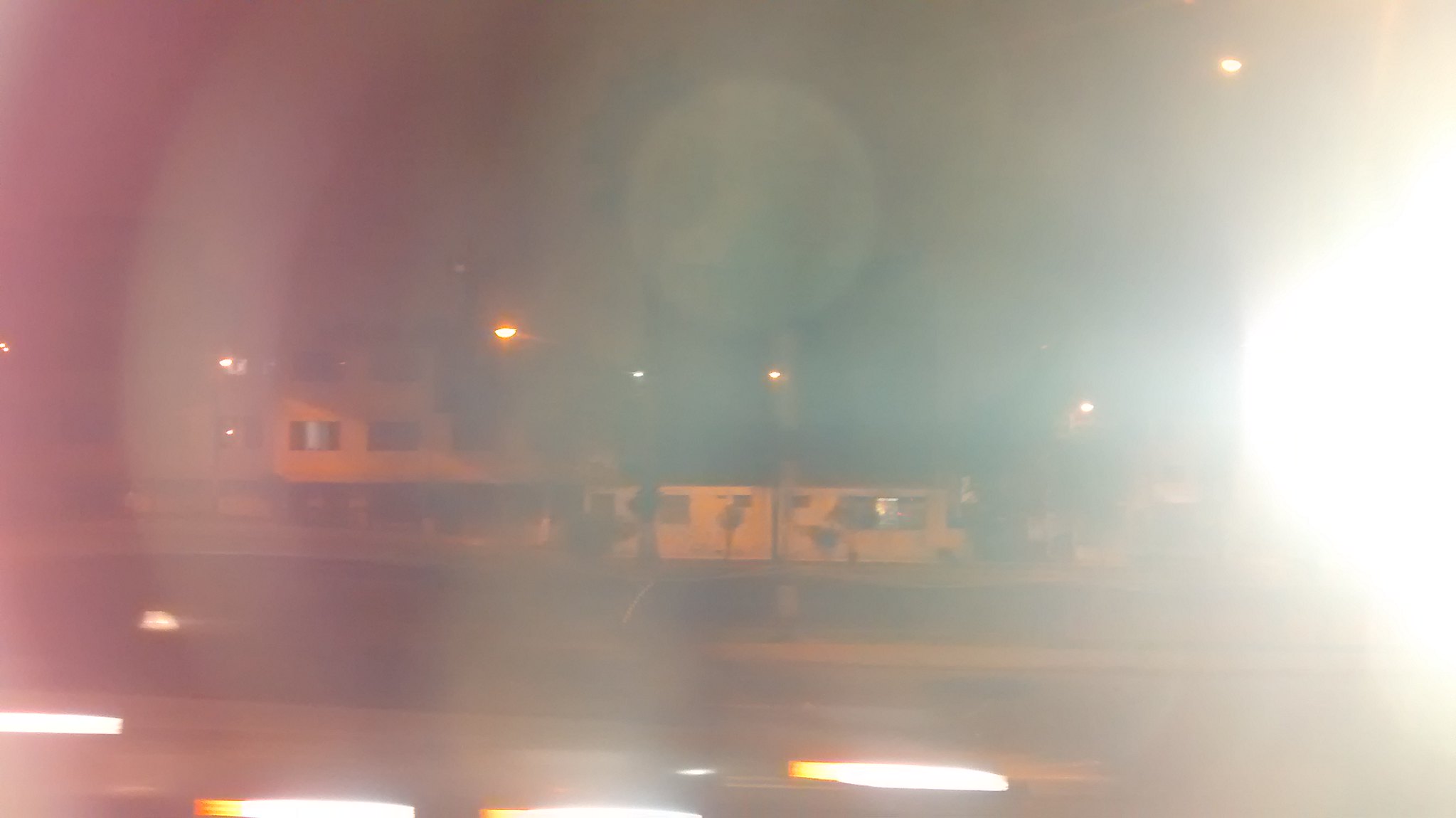The nighttime photograph captures an outdoor urban scene, dominated by a considerable glare from a bright light on the right side, which gives the image a hazy and somewhat blurry quality. Despite this, a few details are discernible. The scene includes a roadway, potentially a busy street, lined with several streetlights and the approaching headlights of a vehicle near the bottom of the image. Across the roadway, there is a large, multi-story building, which appears light-colored and possibly yellow. This building might be part of, or adjoined to, another structure with a similar color scheme. In the background, the moon is visible in the sky, providing additional illumination. Signs of a typical neighborhood are present, suggesting residential homes dotting the landscape, blending together due to the light and blur. An architectural detail noticed includes a gable roof and a window with shutters, possibly indicating one or more houses with lights on inside.